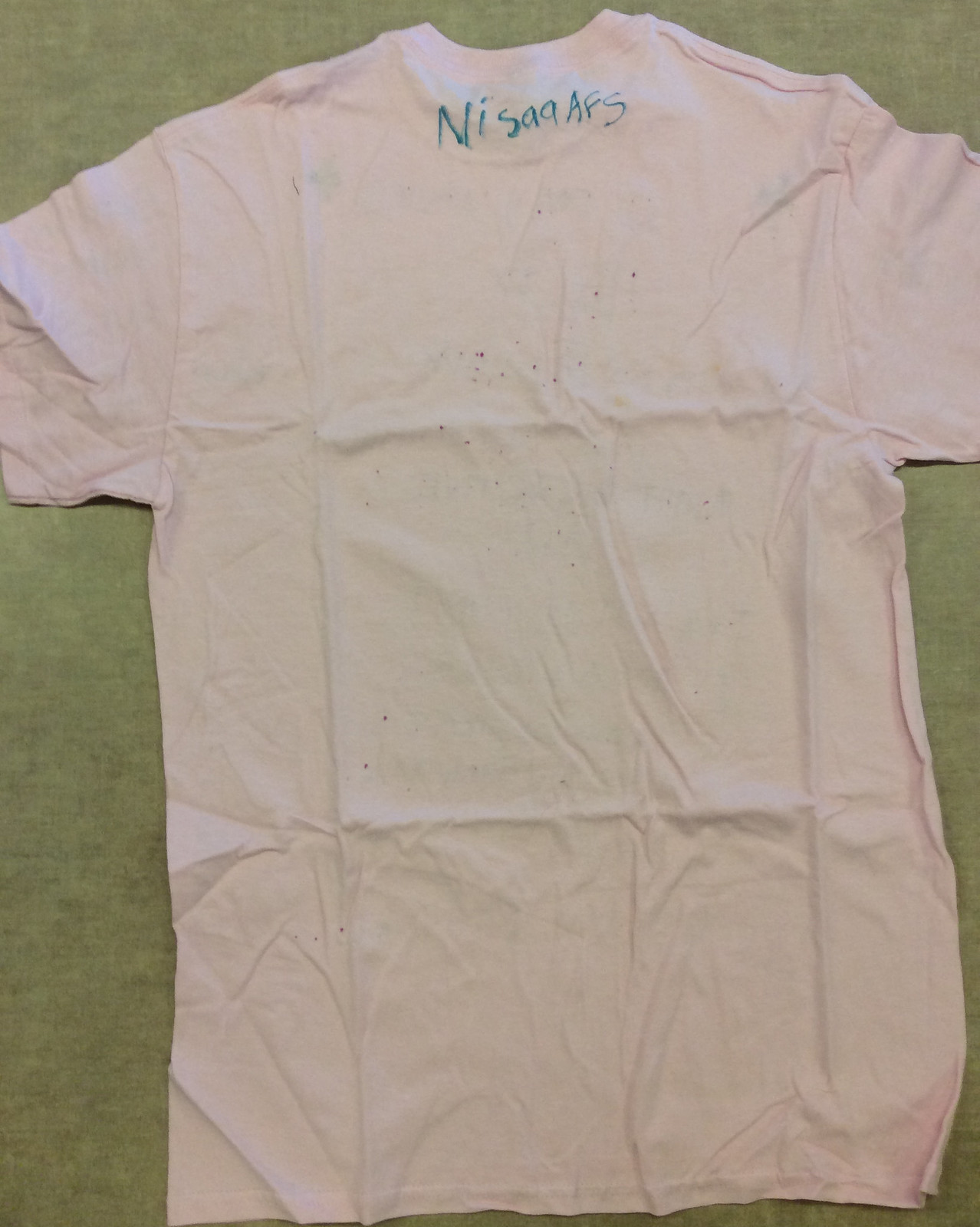This photograph showcases a pale pink t-shirt prominently displayed on a light gray surface, which may contain some shadowy smudges. The t-shirt, viewed from the back, is notably wrinkled and creased, indicative of being folded for an extended period. Sharp, square fold lines are visible alongside more irregular creases. The surface on which the t-shirt rests appears textured, resembling a mix of light and dark gray or a very light tan carpet. At the top of the shirt, near the collar area, there is a written inscription in blue marker ink: "NISAA" in a mix of capital and lowercase letters, followed by "AFS" in uppercase. This image focuses solely on the t-shirt and its immediate surroundings, emphasizing its folded and worn state.